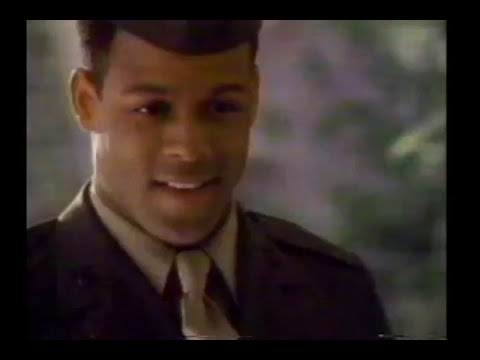This image captures a young African American man in his early 20s, dressed in a dark brown military uniform of what appears to be an army soldier, standing outdoors. He has short, neatly cut hair with a bit of shadow around his jawline, indicating a slight mustache and beard. His uniform includes a matching brown cap and a neatly tied white shirt with a white tie beneath his coat. The man is depicted with a subtle, hopeful smile that reveals some of his teeth, and he has a straight nose with thick eyebrows. The setting behind him is a bit blurry, filled with green leaves and foliage interspersed with grey areas, possibly indicating a garden or an outdoor home environment. The photograph itself has a slightly blurred quality, giving the sense that it might be a still from a film or a television show. The young man's soft, open expression hints at a moment of calm and anticipation, possibly suggesting he's returning home or awaiting someone.